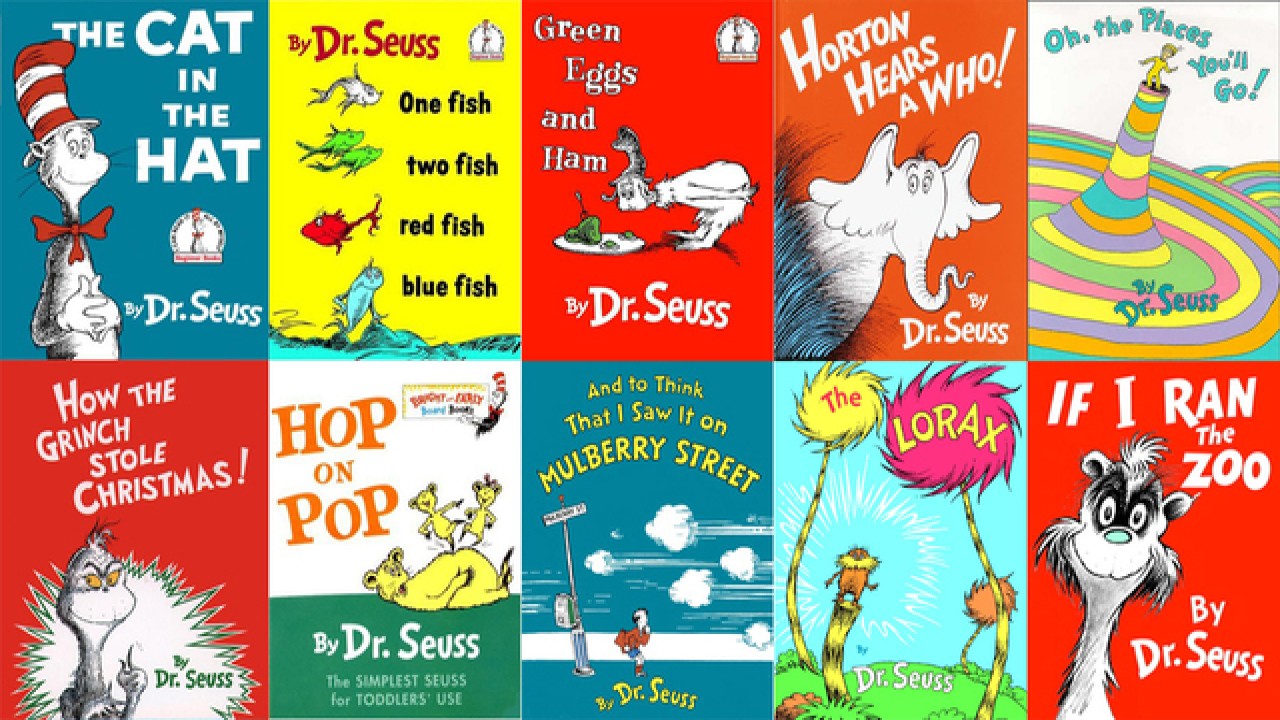The image displays a rectangular arrangement of ten classic Dr. Seuss book covers, divided evenly into two rows. Each book cover retains its iconic design, vividly capturing the essence of Dr. Seuss's beloved stories. 

In the top row, starting from the left:
1. **The Cat in the Hat**: Featuring the mischievous cat with his tall, white and red striped hat and red bow tie against a blue background.
2. **One Fish, Two Fish, Red Fish, Blue Fish**: This yellow-covered book showcases colorful fish in various hues.
3. **Green Eggs and Ham**: The bold red cover with white print prominently displays the peculiar green eggs and ham.
4. **Horton Hears a Who!**: Picturing Horton the elephant on a red background.
5. **Oh, the Places You'll Go!**: A white cover adorned with a multi-colored spiral resembling a whimsical mountain, topped with a small yellow figure.

In the bottom row, from left to right:
1. **How the Grinch Stole Christmas!**: A red cover depicting the Grinch in white.
2. **Hop on Pop**: Featuring a dual-tone cover with a white top half and green bottom half, where a yellow bear and his cubs play.
3. **And to Think That I Saw It on Mulberry Street**: A blue cover with a character dressed in red and blue, observing something zipping by, leaving white smoke trails.
4. **The Lorax**: Showcasing a blue sky and green ground, spotlighting the small, orange Lorax standing by a curious tree.
5. **If I Ran the Zoo**: The final red cover featuring a whimsical white creature, beaming at viewers.

All covers are depicted in bright, engaging colors, characteristic of Dr. Seuss's appeal to children.